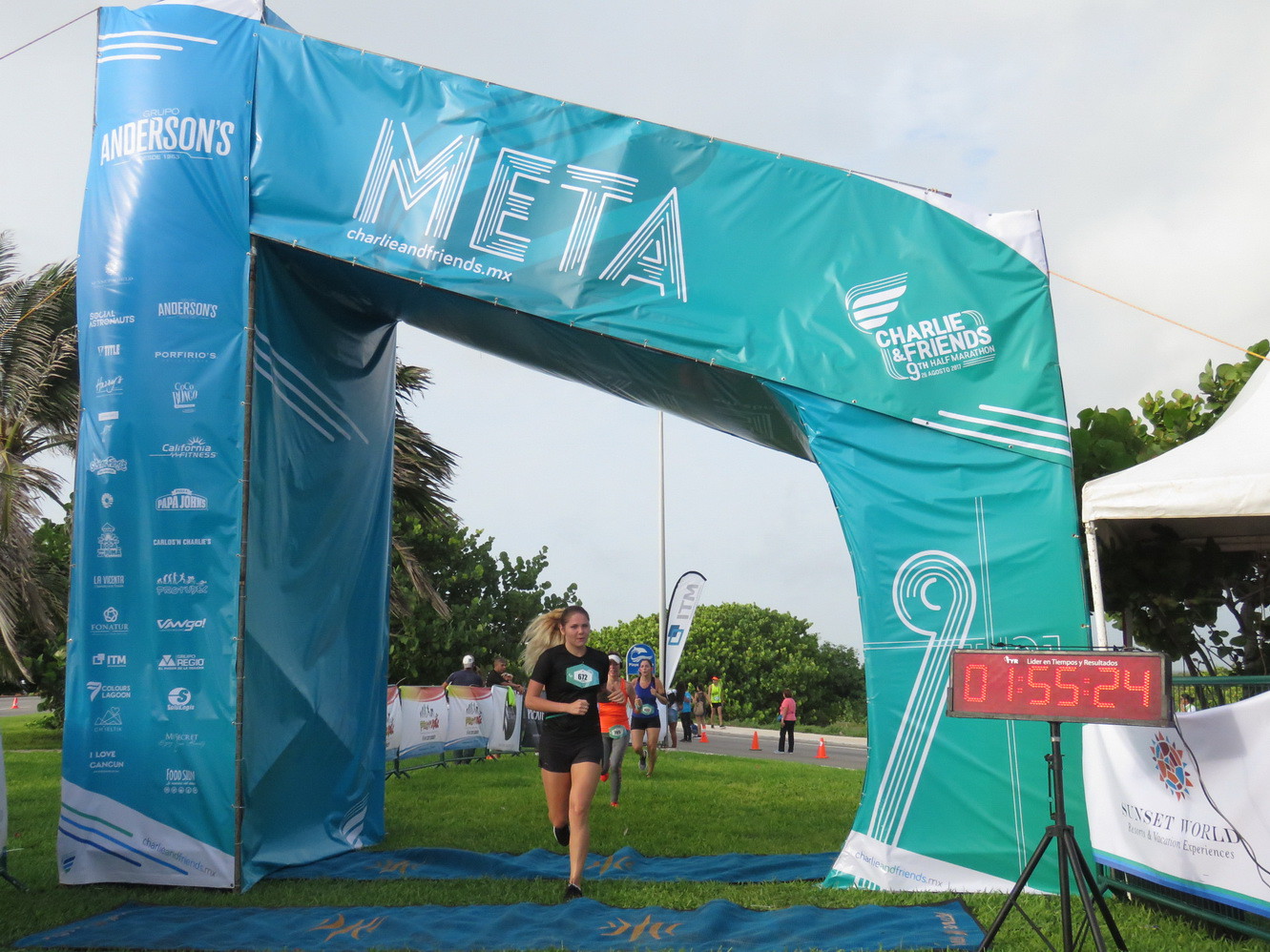The image captures the end of a marathon race set in an outdoor, grassy field. Dominating the foreground is a turquoise blue finish line arch with various sponsor logos, including "META" written at the top in white and blue lettering. A blonde woman wearing a black top with an emblem, black shorts, and dark running shoes is seen sprinting toward the finish line, her ponytail streaming behind her. Just behind her, two other female runners are visible: one in an orange sleeveless top and grey pants, and another in a blue vest and black shorts. Each runner has a race number attached to their attire.

The ground is dotted with blue carpets and several towels. To the right, there's a red digital timer display reading "01:55:24." In the background, palm trees accentuate the tropical feel, while a small white tent featuring a multicolored logo and the words "Sunset World" can be glimpsed. The field is further adorned with various banners, a light post, and traffic cones, adding to the race-day atmosphere. The sky above is mostly overcast, filled with clouds. The image's vibrant color palette includes shades of blue, red, light red, black, white, turquoise, green, yellow, orange, and pink, enhancing the lively and energetic scene.